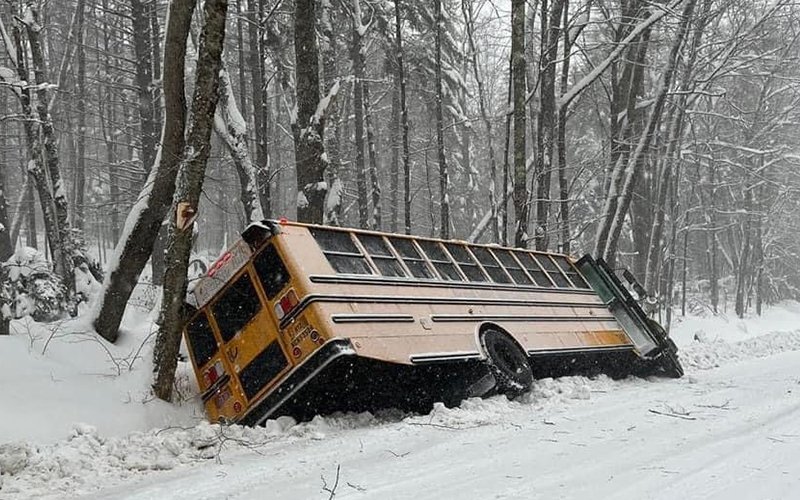In the image, a yellow school bus has skidded off a snowy road and is tilted dramatically on its side in a ditch, possibly at an angle less than 45 degrees. The collision with a tree, situated behind the bus, prevented it from venturing further into a dense, snowy forest. The bus’s door is open and pointing upwards towards the sky, with windows lining its side, though the interior remains dark and obscured. The entire scene is blanketed in thick snow, creating an atmosphere of eerie silence typical of freshly fallen snowfall. The bus rests amid an expanse of white, with brown, leafless trees, heavily laden with snow, populating the background, suggesting a recent or ongoing heavy snowfall in this secluded forest area.